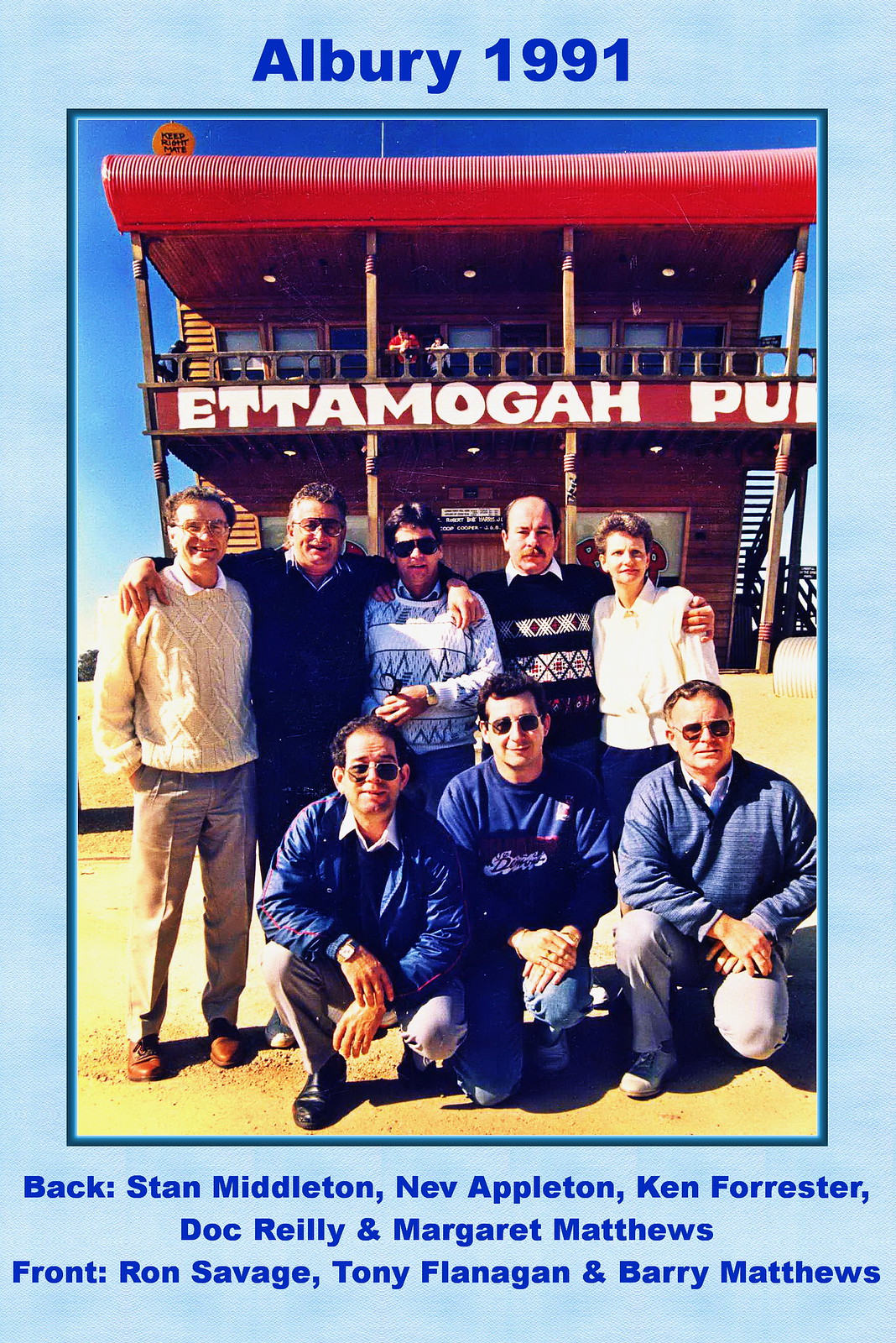This tall rectangular image features a framed photo set against a textured light blue background with a darker blue inner frame. The frame is noticeably thin on the sides and thicker at the top and bottom. At the top in dark blue font, it reads "Albury 1991," and below the photograph, the same dark blue font lists the individuals: "Back: Stan Middleton, Nev Appleton, Ken Forrester, Doc Riley, and Margaret Matthews. Front: Ron Savage, Tony Flanagan, and Barry Matthews." The photograph captures eight individuals posing in two rows; the front row shows three men kneeling on one knee, while the back row has four men and one woman standing. They are positioned in front of a rickety, two-level establishment called Etamogah Pub, identified by large white letters on a red roof, which partially reads "Ettamogah Pub." The building features a balcony, stairs on the right, and appears to be situated in a sandy, beach-like environment with no other buildings in sight. The background reveals a bright blue sky, enhancing the outdoor daylight setting. The men in the back are detailed with different appearances: one in a knit sweater and glasses, another in sunglasses with his arms around others, a man in a patterned sweater, another with a big mustache and a black sweater, and finally a woman in a white blouse. The men in the front all wear blue tops and light-colored slacks, with one distinctively in blue jeans.